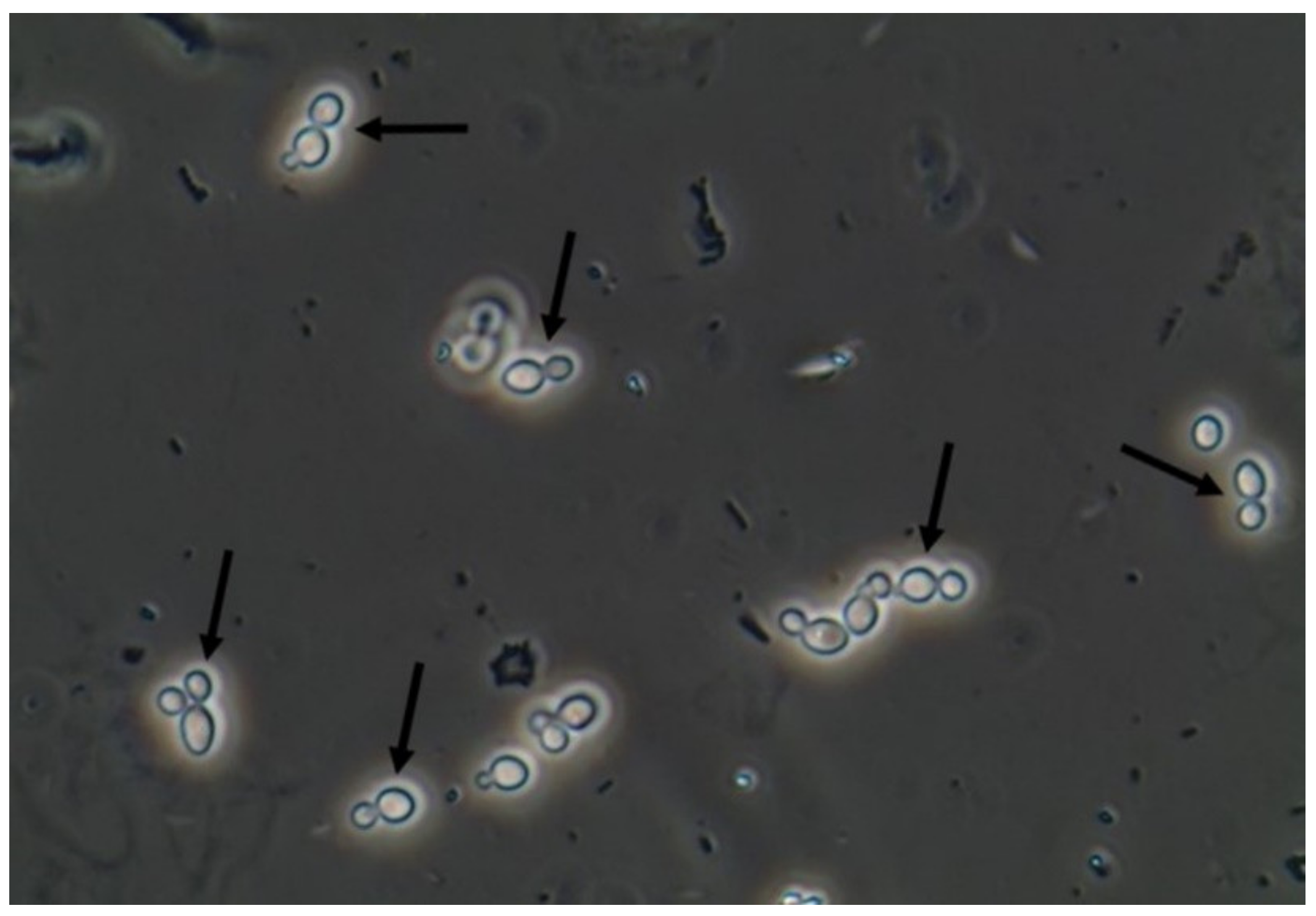In the image, we observe a horizontally aligned rectangular scene that resembles what is typically viewed under a microscope. The backdrop is a dark, brownish-gray hue, speckled with black dots and marked by various indentations resembling circles. Black arrows direct attention to numerous illuminated objects scattered across the field. Positioned predominantly in the bottom half, these objects primarily consist of small, interconnected black round shapes, each encircled by a luminous halo and containing light brown centers.

Several of these formations appear as "figure eights," highlighted dramatically with a white light. One such "figure eight" sits prominently in the upper left, with an arrow pointing to its center. Moving downward, another sideways figure eight is similarly marked. In the middle-left region, there's a shape mimicking paw prints, featuring an oval base and topped with two smaller circles. Nearby, a longer chain of six links extends towards the middle right section. The far right of the image features another distinct "figure eight."

Notably, the ground mass displays additional visual textures: small black flecks of various forms including dots, narrow rectangles, and seed-like shapes, along with some dark blue splotches, one of which intriguingly looks like a tiny kangaroo facing left, located just below the top middle edge. Together, these details create a complex and glowing tapestry of interconnected structures under a dark, speckled background.